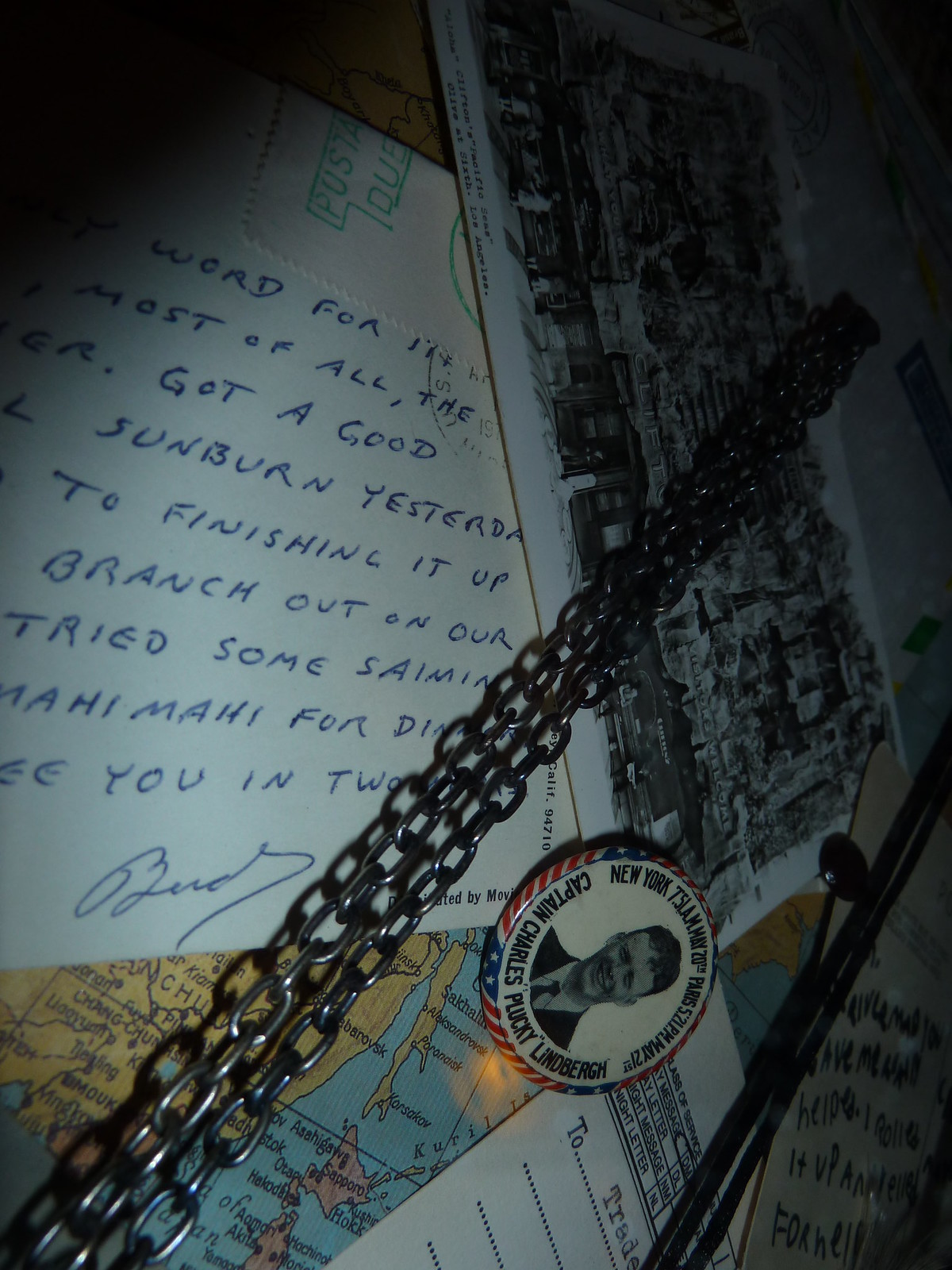The image features a slightly canted view of a bulletin board or a similar background. At the bottom left corner, a chain with three rows or columns extends diagonally to the top right, creating an unusual visual effect. To the left of the chain, there is a slightly worn sheet of paper with blue ink and a partial signature at the bottom. The legible text mentions, "got a good sunburn yesterday," and continues with fragmented phrases such as "finishing it up, branch out on our tried, some, same," and a few other incomplete sentences. On the right side, there is a thicker, black and white picture that might be a book or magazine cover, primarily composed of dark shapes. Below these items sits a round badge featuring a gentleman's face, surrounded by text reading "New York, Tsunami, Press," though some of it is too small to decipher. The badge names "Captain Charles Lindbergh" within a red, white, and blue ring decorated with stars.